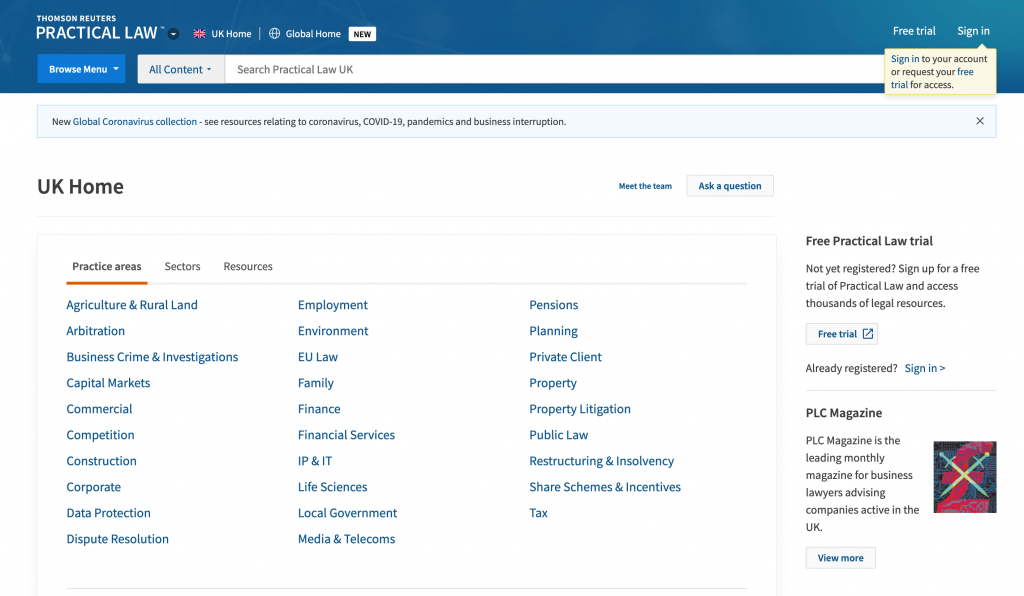The webpage displays a prominent blue bar at the top with a message that reads, "New Global Coronavirus Collection: See resources relating to coronavirus, COVID-19, pandemics, and business interruption." Directly below this banner, the top of the page features a navigation label reading "UK Home." The central part of the webpage includes a categorized box with selectable tabs labeled "Practice Areas," "Sectors," and "Resources." The "Practice Areas" tab is actively selected, showcasing a meticulously organized list of practice areas in three columns. Examples from this alphabetical list include "Agricultural and Rural Land," "Capital Markets," "Construction," "Family," "Life Sciences," "Property," "Litigation," and "Public Law," indicating specialized legal fields. Adjacent to this list, in a right-hand sponsored column, there is an advertisement promoting a "Free Practical Law Trial" alongside a mention of "PLC Magazine." The layout suggests a resourceful interface aimed at providing legal professionals with streamlined access to subject matter expertise and practical legal resources.